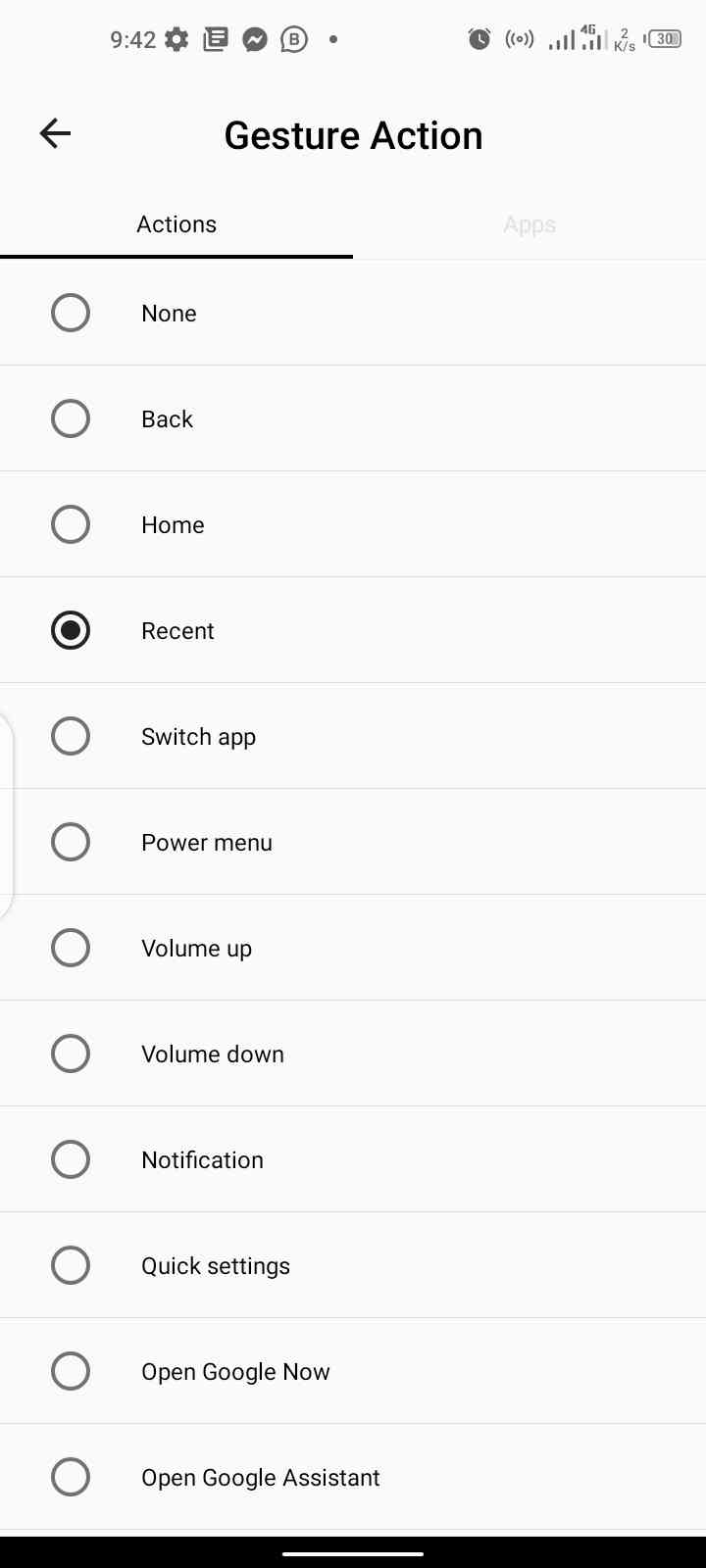A user is navigating the "Gesture Action" settings on an Android phone. The screen displays two tabs at the top labeled "Actions" and "Apps." The "Actions" tab is currently active, showing a list of gesture options, each accompanied by a radio button, allowing for single selection. The available gesture actions include: "None," "Back," "Home," "Recent," "Switch App," "Power Menu," "Volume Up," "Volume Down," "Notification," "Quick Settings," "Open Google Now," and "Open Google Assistant." The radio button next to "Recent" is selected, indicating that a specific gesture is set to open the Recent Apps view. Although the specific gesture isn't indicated, it can be changed to any of the other listed options. The interface is set against a light gray background. The notification area at the top of the screen shows icons for various active alerts, including an alarm.